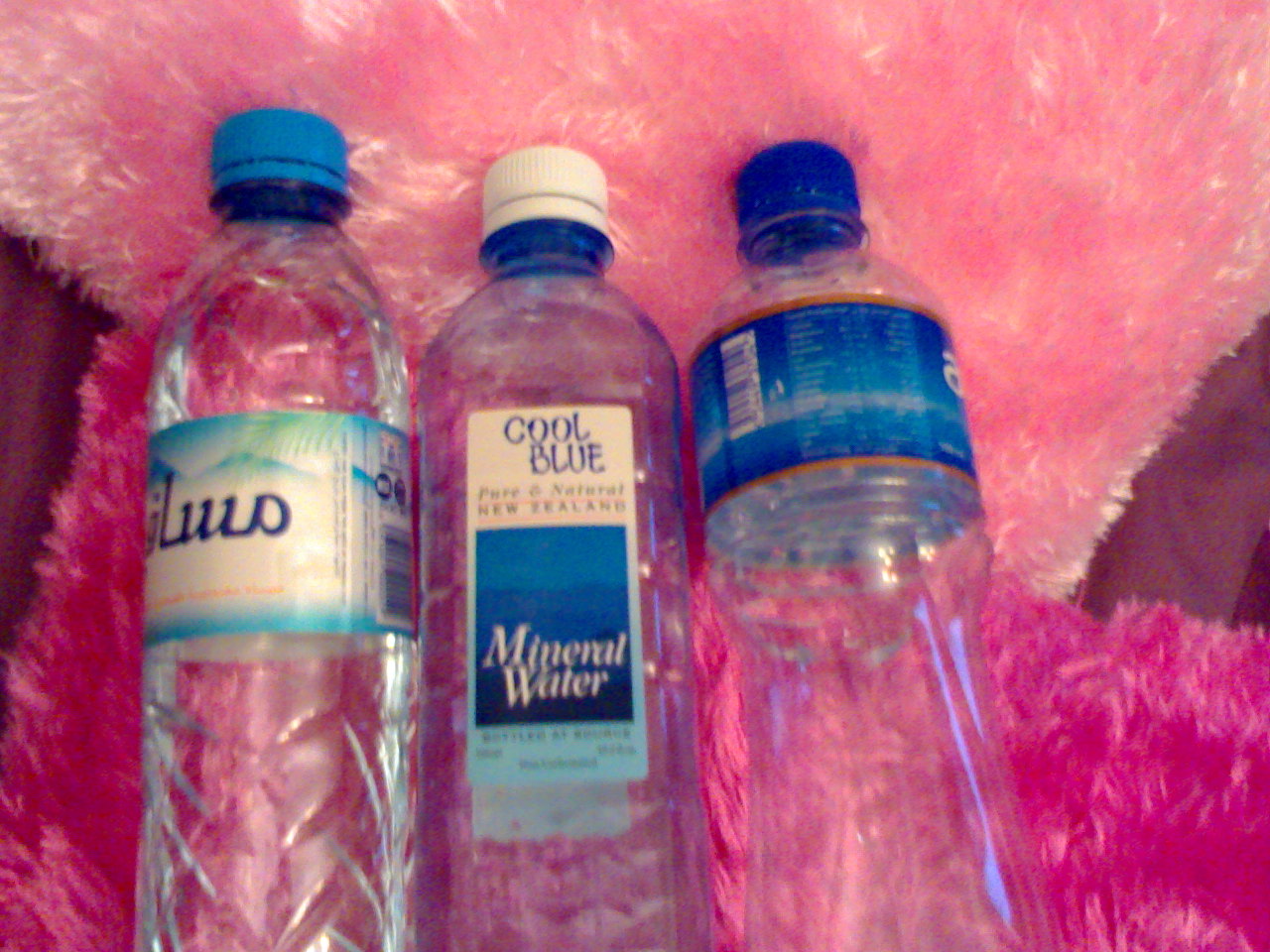The image depicts a slightly blurry photograph of three distinct plastic water bottles arranged on a surface adorned with two fluffy, pink pillows. The pillows add a vibrant backdrop with one being a bright, furry pink and the other a lighter rose pink hue. The water bottles are positioned in the center of the image, with each bottle featuring different designs and labels. On the left, the bottle with a white and blue label ending in the letters "L-I-U-O" has a blue cap. The middle bottle, with a white cap, prominently displays the words "cool blue" and "mineral water" on its white and blue label, including a hint of light teal at the bottom. The bottle on the right, adorned with a blue label accented by gold at the top and bottom, also has a blue cap. Despite the varied orientations of the bottles making some labels difficult to read, each stands out against the contrasting pink, fuzzy background, likely a wooden table layered with the pink pillows.